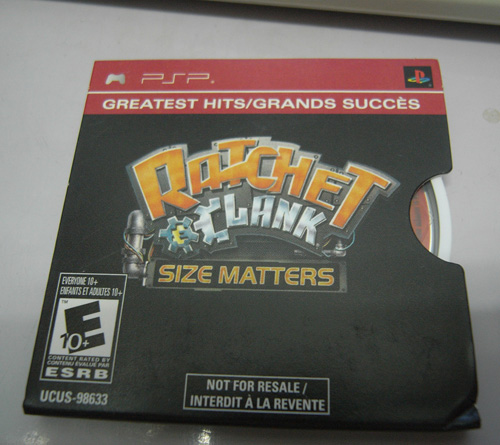The image is of a PSP (PlayStation Portable) game cover for "Ratchet & Clank: Size Matters" resting on a hard white surface. The cover features a bold red banner at the top, prominently displaying the PSP logo next to the text "Greatest Hits / Grand Success." The primary colors of the packaging are black and red, with text in white, black, golden, and silver. The title "Ratchet & Clank: Size Matters" is printed in eye-catching 3D yellow and silver fonts. Below the title, the cover indicates that the game is rated E10 by the ESRB, suitable for everyone aged ten and up. A section at the bottom reads "Not for Resale / Interdit à la revente," highlighting its status as a special edition likely included as a promotional pack-in with PSP consoles rather than a separate retail item. The disc is slightly poking out from the side of the cardboard case, which features a cutout area designed for easy access. There is no specific release date or additional context provided within the image.